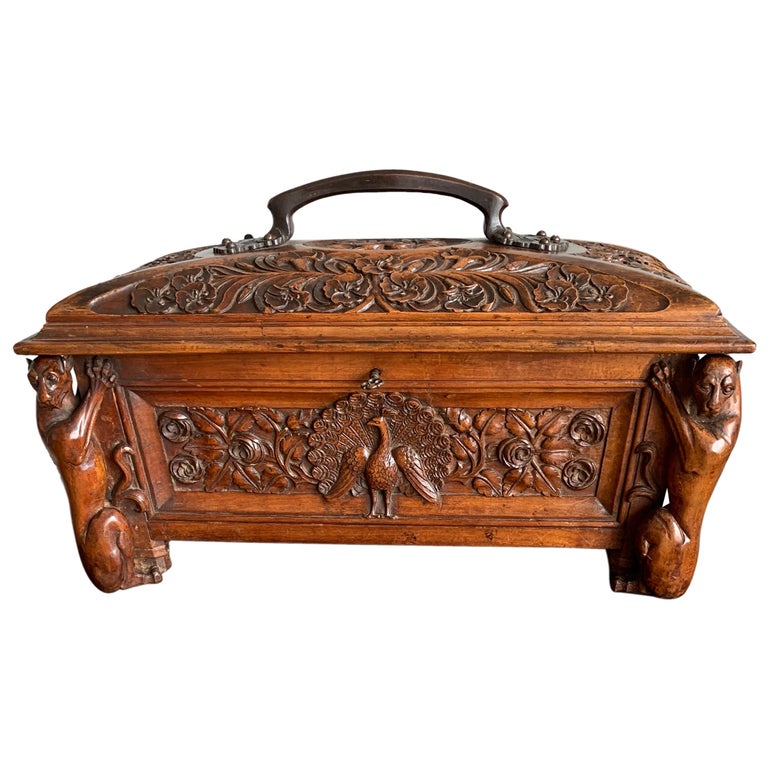This is a horizontal, borderless image depicting an ornate wooden chest, characterized by its richly detailed carvings and intricate design. The chest is an orange-copper color and features a smooth, tapered edge. The lid is roundish and adorned with an elaborate handle. Intricate floral patterns, including prominent flower buds, embellish the lid. On the front of the chest, a peacock is prominently carved in the center, its feathers majestically spread out. Flanking the peacock, on both the left and right sides, are feline figures, their heads just beneath the tapered lid, seemingly clawing the sides of the chest. The overall design is both opulent and meticulously crafted, creating a visually stunning piece of art.